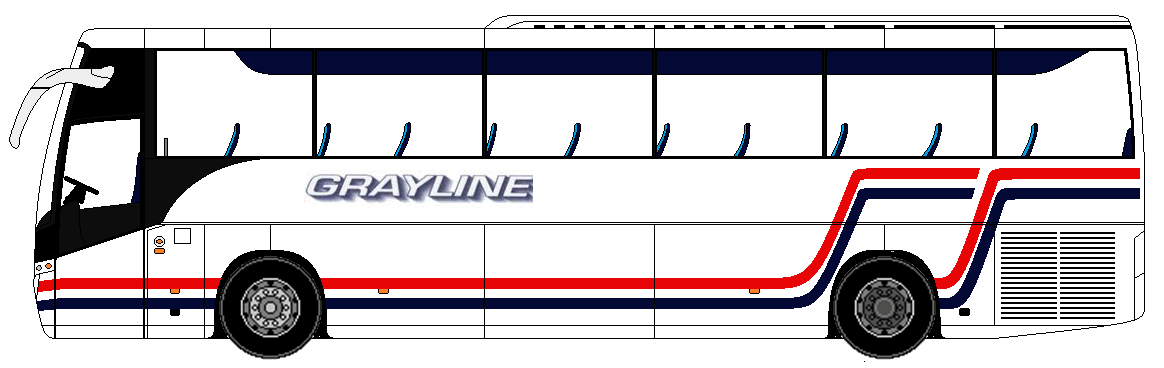The image is a detailed illustration of a modern city or tour bus viewed from the side. The bus features a sleek, elongated body, common for standard single-deck passenger buses. The exterior is predominantly white, accented with a striking pattern of red and blue stripes. Starting at the bottom, a red line runs straight from the front to the back wheel before curving upward just below the windows and then extending straight again towards the back. Another red line begins at the rear wheel and follows a similar path, curving up under the windows before continuing straight. Below these red lines, two dark lines run along the length of the bus.

The logo "Greyline" is prominently displayed towards the front, printed in white text with a grey drop shadow, adding a touch of sophistication to the design. The front section, where the driver’s cabin is located, is framed in black paint, clearly visible through the front window along with the steering wheel. The illustration includes six windows, each revealing at least one seat, emphasizing the bus's capacity for passengers. Overall, the image appears to be a meticulous design diagram, possibly for a specific bus company.